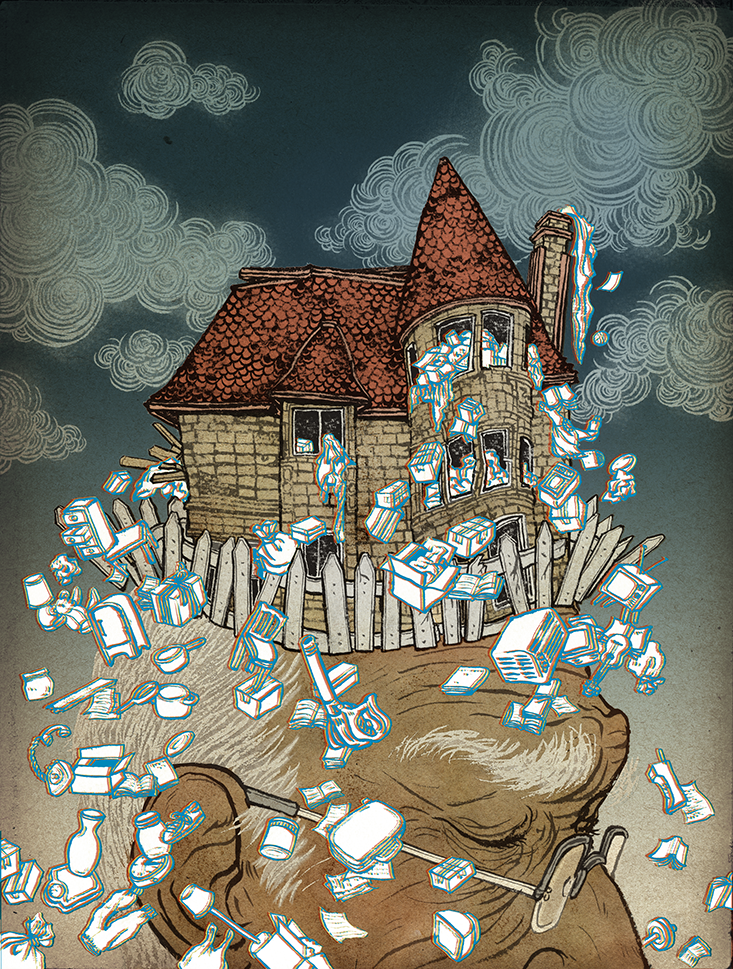This detailed illustration depicts an elderly man with white hair, bushy eyebrows, and glasses, his head tilted down and to the right with closed eyes. Sitting atop his head is a dilapidated three-story Victorian-style house with brown siding and a red tiled roof, complete with a chimney emitting a viscous substance. The house is surrounded by a white picket fence. Strewn around and spilling out of the house are numerous objects, including vases, newspapers, a refrigerator, a chest of drawers, pots, pans, and furniture. The backdrop features a dark sky filled with swirling clouds made up of concentric circles.